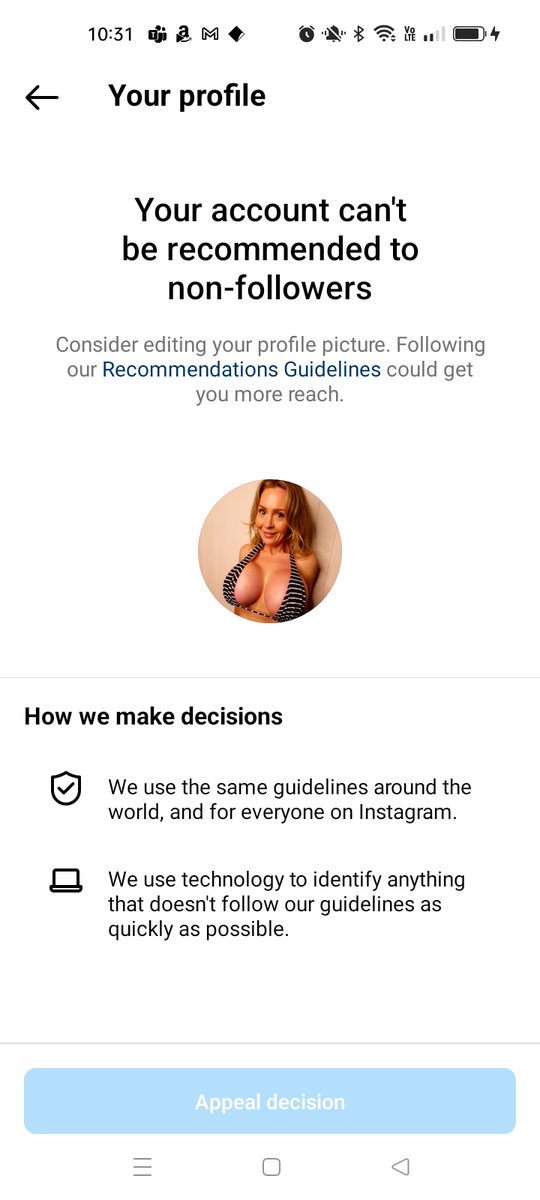The image captures an individual's attempt to create an Instagram account using a controversial profile picture. The profile picture in question is a self-portrait of a woman with large breasts. Instagram's guidelines seem to have flagged the image, preventing her profile from being recommended to non-followers. The platform's message indicates that her account is restricted, suggesting she consider editing her profile picture. The notification states: "Your account can't be recommended to non-followers. Consider editing your profile picture." 

Instagram's decision appears to have come after a review process and is explained in the notification: "We use the same guidelines around the world and for everyone on Instagram. We use technology to identify anything that doesn't follow our guidelines as quickly as possible." 

At the bottom of the notification, there is a light blue button labeled "Appeal Decision," offering the option to challenge the ruling.